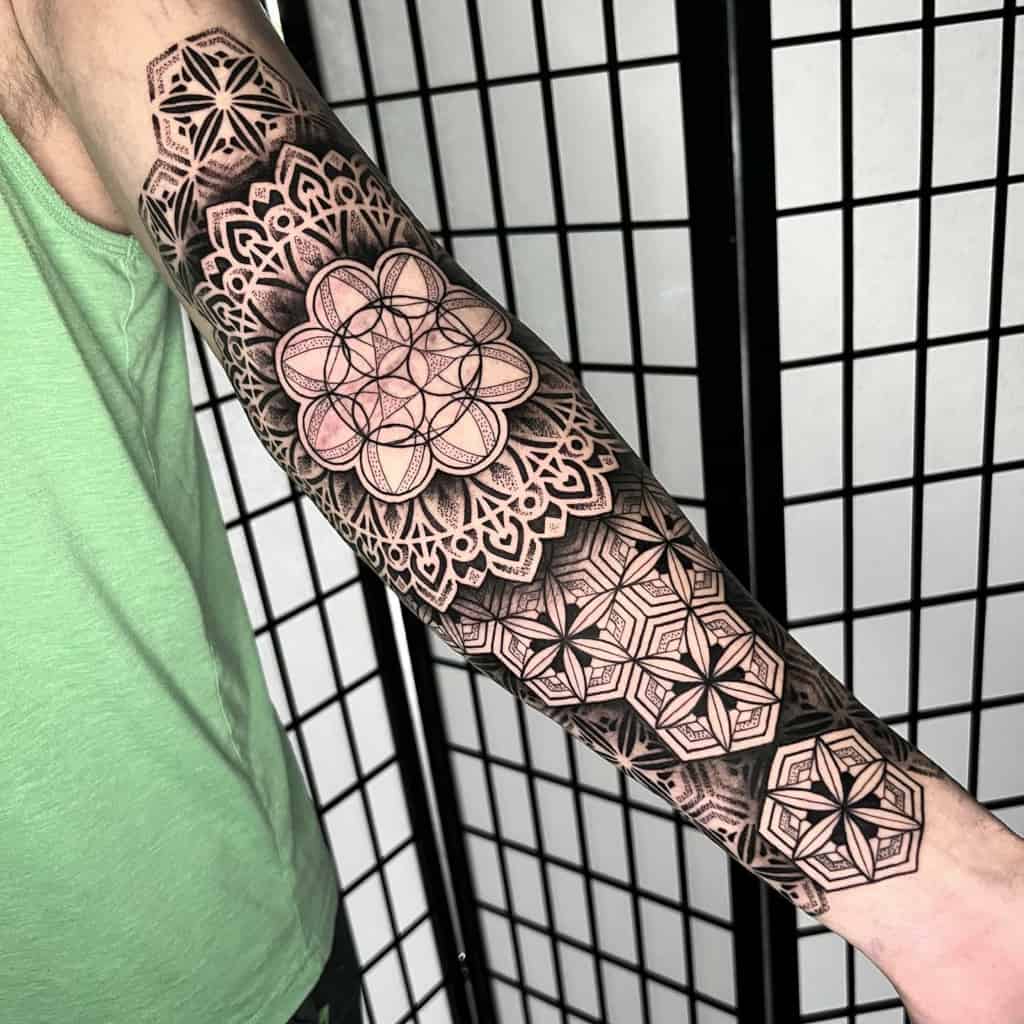The photograph captures a man's arm, extended diagonally from the top left to the bottom right corner of the image, adorned with a fresh, intricate black tattoo. The detailed design features symmetrical geometric shapes and mandala-like patterns, creating a full sleeve effect from the wrist to the upper arm. The most prominent element of the tattoo is a large, multi-layered floral design centered on the elbow. The man's body, partially visible on the left edge of the frame, reveals him wearing a light minty green shirt, with a hint of armpit hair at the top left corner. His skin appears pinkish, possibly indicating the recent completion of the tattoo. The background features an oriental, black and white accordion folding screen, suggesting the setting is likely a tattoo parlor.